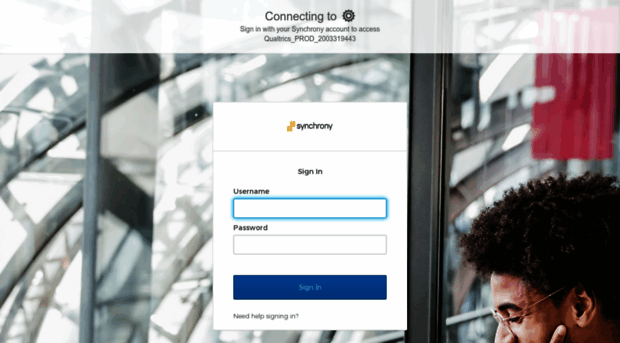The website screenshot features a semi-transparent white banner at the top overlaying a background image, allowing the background to remain partially visible through the frosted effect. Centrally, the banner displays text stating "Connecting to," followed by a sun-like graphic. Adjacent to this, the text reads: "Sign in with your Synchrony account to access Qualtrics." Below this text, a string appears: "_PRCO_2003319443".

The background image depicts a building with architectural elements, including a circular feature and a straight bar. On the right side, barely visible from the nose up, is the left side profile of a man's face.

In the center of the screen, a prominent square section contains the website’s login interface. At the top is the Synchrony logo, featuring two small gold squares beside the name "synchrony," written in lowercase letters. Below this is the word "Sign in" with a capital S, followed by fields for "Username" and "Password" which has a turquoise border around the username field. At the bottom is a blue button labeled "Sign In." Lastly, below the button, there is a link stating "Need help signing in?" with a question mark.